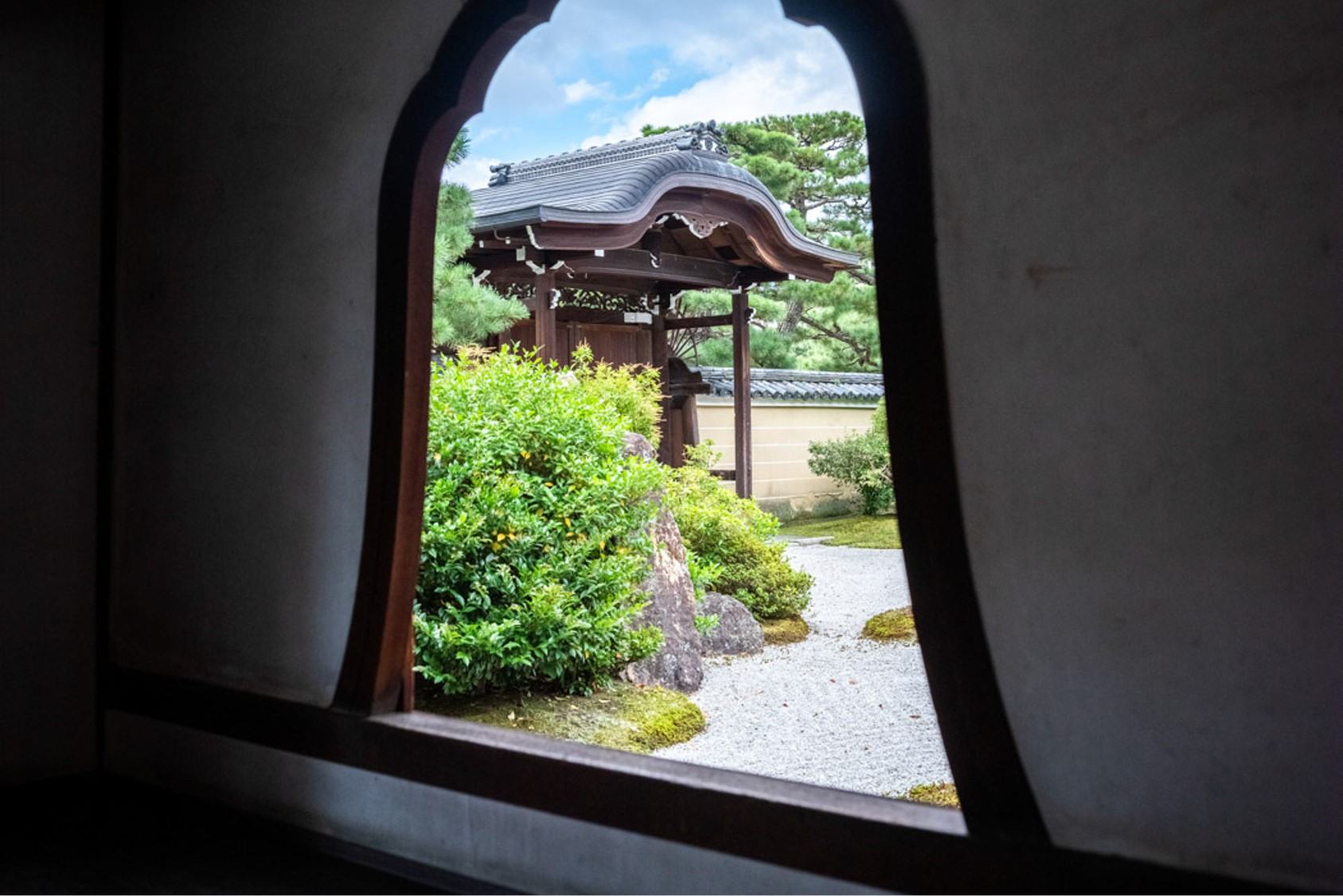This photograph captures an outdoor scene viewed through a bell-shaped, arched window with dark brown wooden trim, set in a white, possibly slightly dirty, wall. The image reveals a beautifully landscaped garden featuring a dark-colored, wooden Chinese-style structure adorned with intricate carvings on its black roof and supported by wooden columns. The foreground showcases a gravel walkway bordered by lush green shrubbery and stones, leading the eye towards the structure. To the right of the scene, decorative trees and grass add to the garden's serene atmosphere. In the background, a light tan stone wall topped with black ceramic tiles runs across the frame, while large, vibrant trees stand behind it against a bright blue sky dotted with white clouds. This picturesque setting evokes the tranquil ambiance of a traditional eastern garden, possibly Japanese or Chinese.